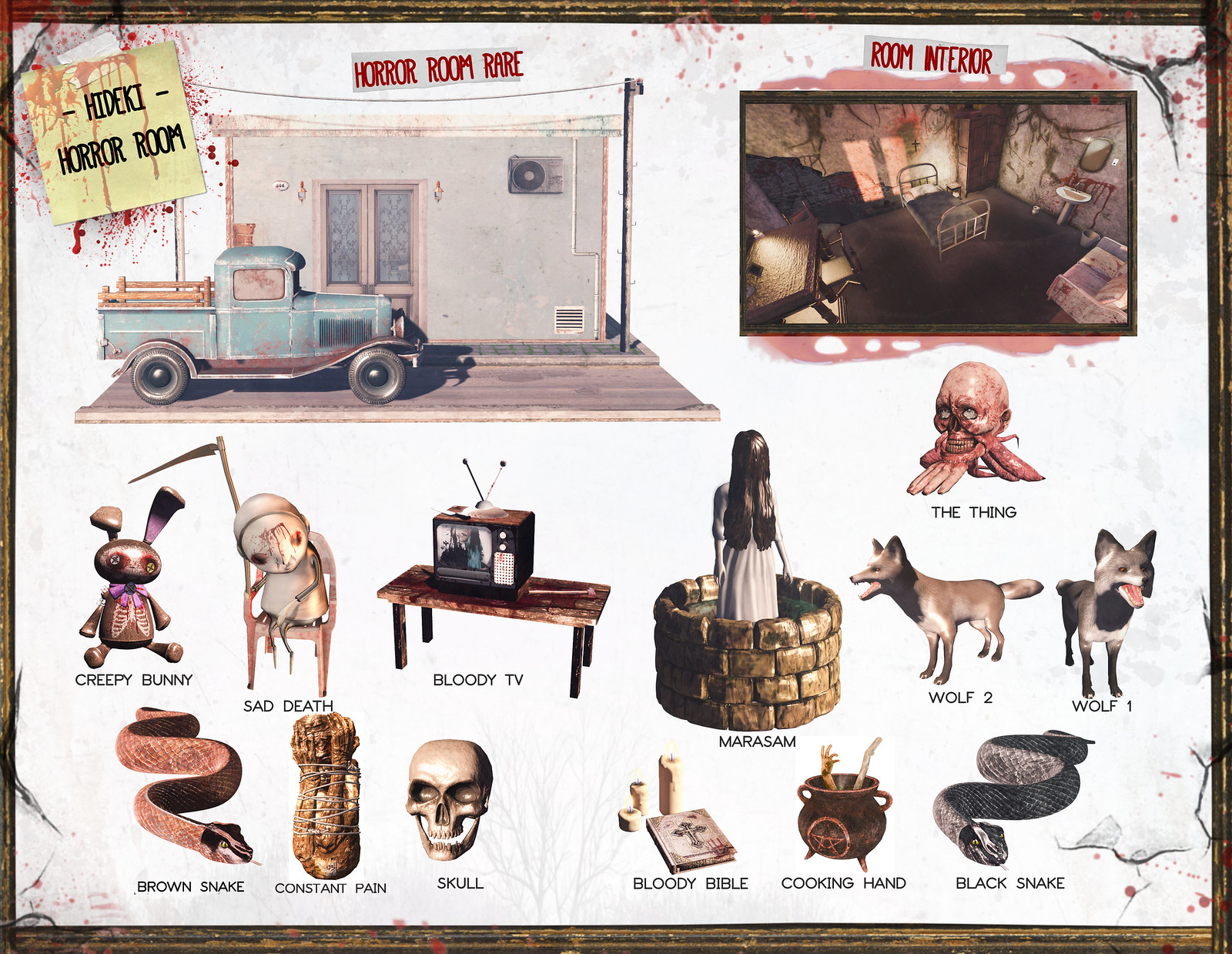This poster, bordered by a black trim resembling wood, showcases an eerie, animated scene reminiscent of a video game. The poster is predominantly white and features various grim images. 

In the upper left corner, a yellow sticky note with blood splatters reads "HIDEKI HORROR ROOM" in black letters, beneath which "HORROR ROOM" is inscribed. To the right, a long rectangular banner declares "HORROR ROOM RARE" in red capital letters, positioned above a depiction of an exterior building facade with a telephone wire overhead. An old-time, pale bluish pickup truck with wooden rails is parked in front.

Further right, another rectangular tape at the top marks "ROOM INTERIOR." The image beneath this label depicts a dark and dingy bedroom with a single bed, a simple brown desk, and a single sink, all stained with blood. The reflection of what looks like two windows can be seen on the wall.

The bottom half of the poster contains a collage of macabre items labeled with text and visuals. This includes:
- A gory head labeled "THE THING"
- "CREEPY BUNNY"
- "SAD DEATH"
- "BLOODY TV" accompanied by an image of a bloody television
- "MARISAM," showing a girl in what appears to be a well
- "WOLF 2," a picture of a wolf
- "WOLF 1," a darker wolf
- "BROWN SNAKE"
- "CONSTANT PAIN," depicting a person tightly wrapped in fishnet
- "WHITE SKULL"
- "BLOODY BIBLE"
- "COOKING HAND," featuring a vat with a hand hanging out
- "BLACK SNAKE"

The detailed illustrations suggest that these graphic elements are parts of a video game or a digitally crafted haunted house experience.